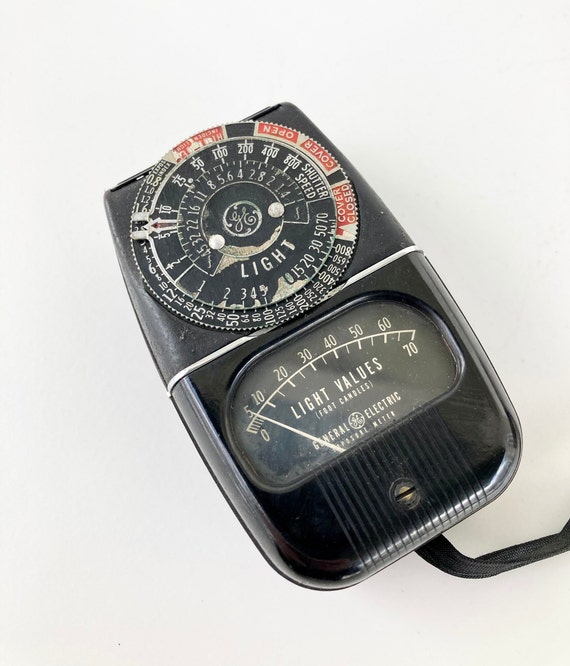The image depicts an old-time General Electric light meter, primarily black in color with various dials and gauges. Central to the device is a circular dial, with numbers ranging from 0 to 70, currently pointing at 5. The light values are denoted around the dial with markings: 45, 32, 22, 16, 11, 8, 5, 6, 4, 2, 8, 2, 1, 4. The outer casing resembles the size of a computer mouse and features both black and metallic elements. In the middle, the device has "GE" with two white dots beside it. Above this dial, red and white text indicates "cover closed," "cover open," and "high." Additionally, there is a metal wheel-like component and various other readings, including ISO and shutter speed values. A cord extends from the bottom right corner of the device, and the entire setup rests on a white background, emphasizing its vintage appearance.